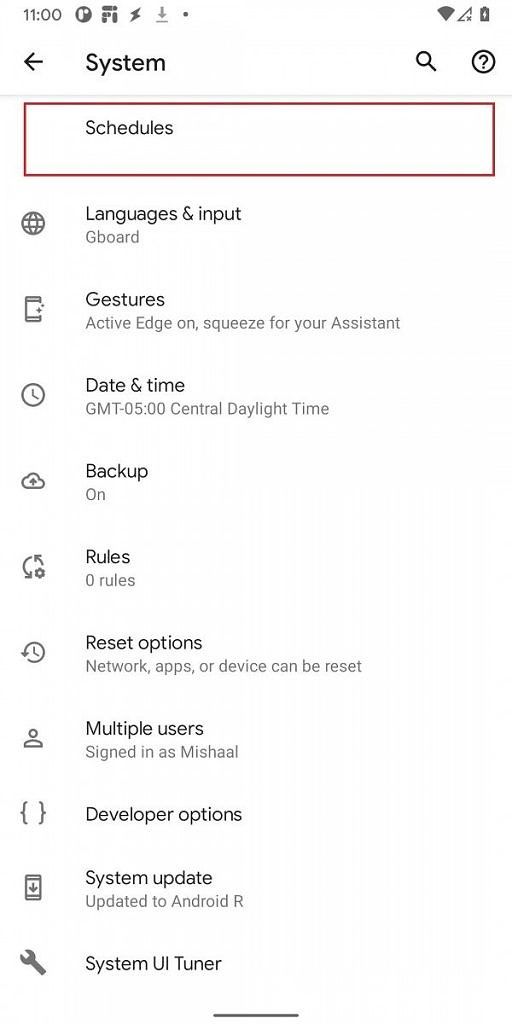Screenshot showing detailed System Settings on an Android phone in Light Mode. The settings menu, displayed against a white background with black text, reveals various options such as "Schedules," "Languages and Input," "Gestures," "Date and Time," "Backup," "Developer Options," and "System Update." Notably, a rectangular red line box has been edited around the "Schedules" option, drawing attention to it. The notification bar at the top indicates no cellular service, as evidenced by an "X" on the reception icon, while the Wi-Fi signal is at full strength. The battery is fully charged and the device is plugged in. This setting screenshot illustrates the extensive customization options available on Android devices, highlighting its greater flexibility compared to iPhones.